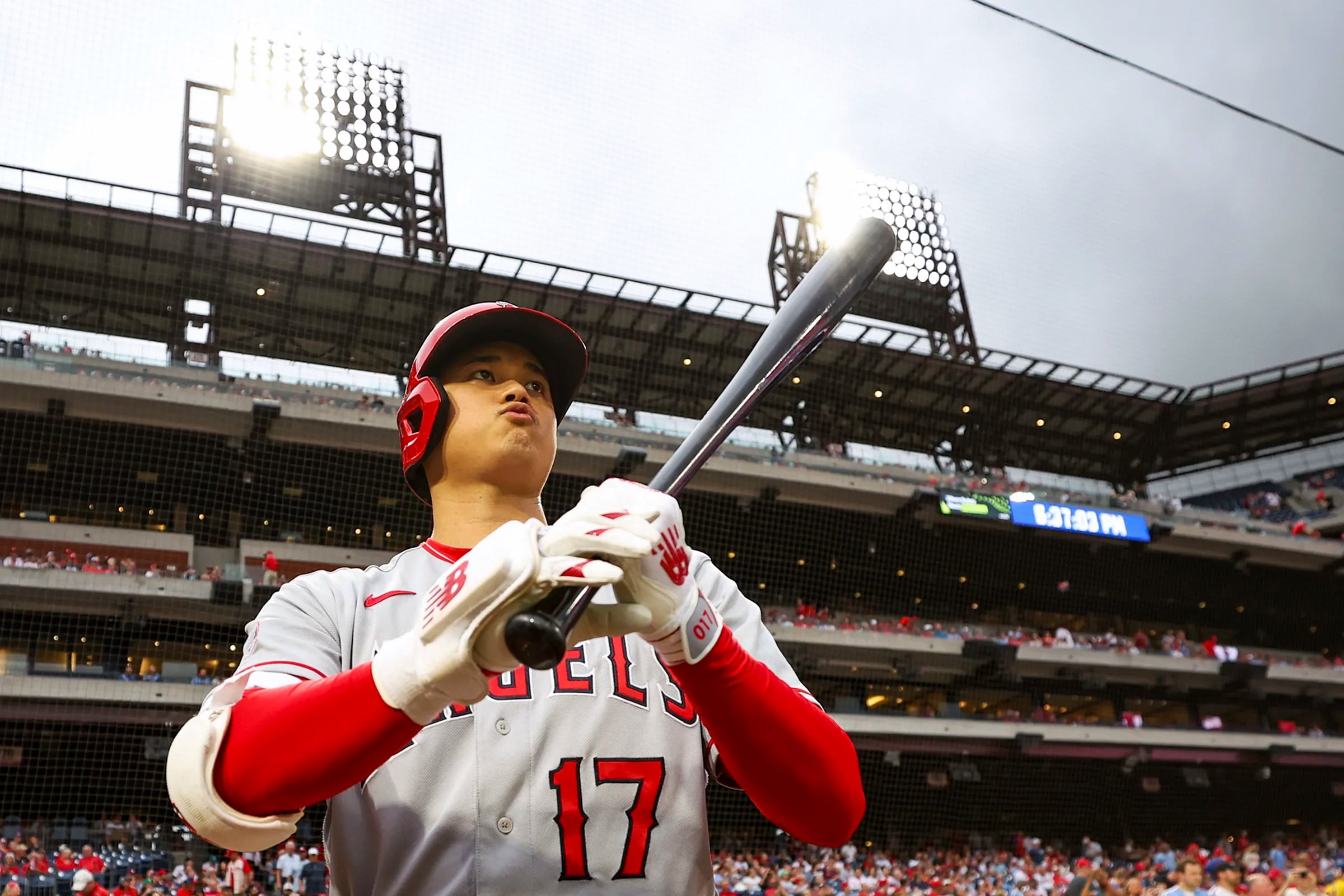This photograph captures a player from the Los Angeles Angels, wearing the number 17 jersey, as he prepares to bat. He is shown in a light gray uniform top with the word "Angels" across the chest and a red long-sleeve shirt underneath. The player is equipped with a red batting helmet, featuring ear protection on his right side, white gloves with red striping and the New Balance logo on the back, and a white elbow pad on his right elbow. Holding a black bat with his right hand beneath his left, he appears focused and determined, pursing his lips as he gazes into the distance.

The image is taken from a low, upward angle, dramatically highlighting the player against the backdrop of a packed stadium. The stands, consisting of four decks filled with fans, suggest a high-energy atmosphere. The stadium lights are turned on, illuminating the scene despite the sky being only partially dark and somewhat overcast. A large square bracket with multiple lights is also visible, contributing to the vibrant ambiance of the night game.